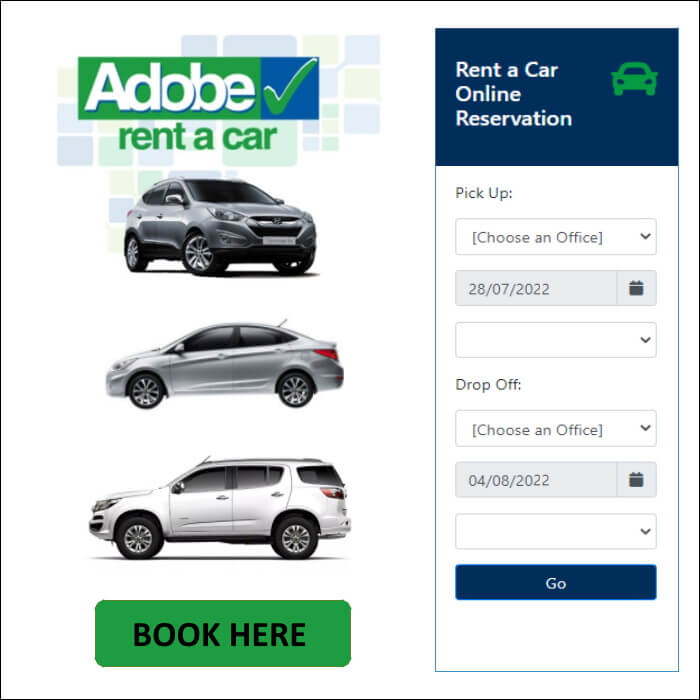This image serves as an advertisement and user interface for Adobe Rent-A-Car, highlighting the online reservation process. 

At the top left corner, the Adobe Rent-A-Car logo is prominently displayed, featuring the word "Adobe" in green accompanied by a check mark. Below the logo are images of three different cars: a silver SUV at the top, a silver sedan in the middle, and a white SUV at the bottom. 

At the lower part of the screen, there's a prominent green button labeled "Book Here" in black text, although the choice of black text on a green background might reduce contrast and readability. 

On the right side of the screen is the reservation form titled "Rent-A-Car Online Reservation," accompanied by an icon of a green car. The form includes a drop-down menu labeled "Choose an Office" to select the pickup location. The pick-up date is set for July 28th, 2022, indicated with a calendar icon. There is also a field to choose a drop-off office and a drop-off date, which is set for August 4th, 2022. 

Overall, the image effectively displays the car rental options and provides a straightforward online reservation form. The use of clear visuals and intuitive form fields enhances user-friendliness and ease of navigation.